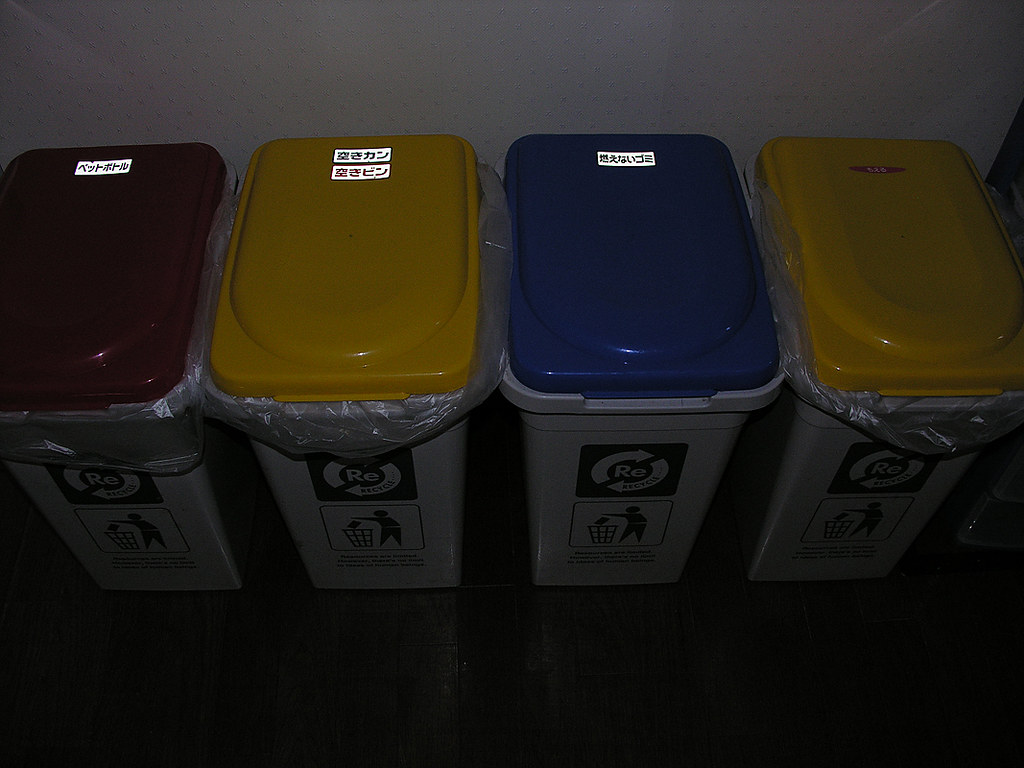The image captures a row of four plastic recycling bins positioned side by side against a white wall, viewed from a slightly overhead angle. Each bin body is grey and features a green square on the front with a white circular arrow and the letters "RE" in the center, accompanied by an illustration of a person tossing trash into a bin. The lids of the bins are distinctly colored: the first bin has a red lid, the second has a yellow lid, the third has a blue lid, and the fourth also has a yellow lid. Printed labels with Japanese script are affixed to the tops of the lids, with some bins displaying multiple stickers in red and green text. Although the surroundings are dimly lit, the lids are notably more illuminated. White plastic bags protrude slightly from under the lids of all the bins except the third one. The bins stand on what appears to be a dark, possibly green or black, floor.